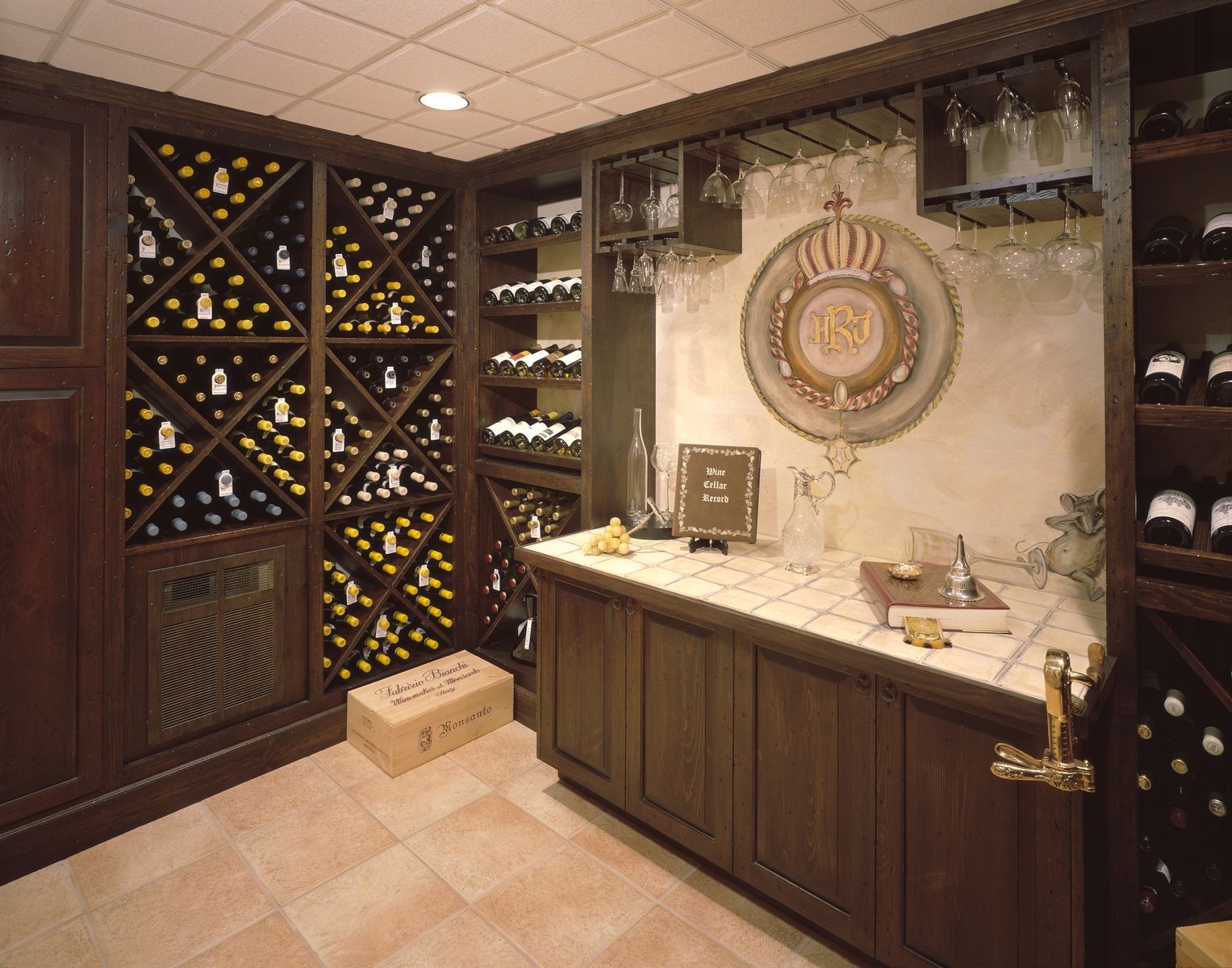This image features a well-organized wine room, potentially situated in a home rather than a commercial space. The room has a cream-colored tile floor with white ceiling tiles, which includes square tiles accented by recessed fluorescent lighting in the corner. The focal point of the room lies along the brown wall to the left, where an intricate storage system for wine bottles is visible. This storage area is composed of X-segmented square sections forming triangles, each holding 12 bottles of wine. The triangles are oriented in different directions, and the bottles within each triangle share the same cork color, categorized into shades of yellow, white, and blue.

To the right of the room, there is a wine bar with a marble-like crust on the wall and tiles on top, where numerous wine glasses hang upside down from shelves, creating a restaurant-like ambience. Below the bar are additional wooden storage compartments holding various bottles of wine. The back wall of the room displays four rows of wine bottles laying on their sides, each row able to hold six bottles.

Other notable details include a box on the floor, several books propped up on a table, and a logo with the letters "HRJ" adorned with a crown. There is also a hanging sign, likely indicating something about a wine cellar record. Additionally, a drawing of a tipped-over wine glass with a mouse is seen on the wall, enhancing the cozy, personalized touch of the wine collection space. No people are present in the scene.